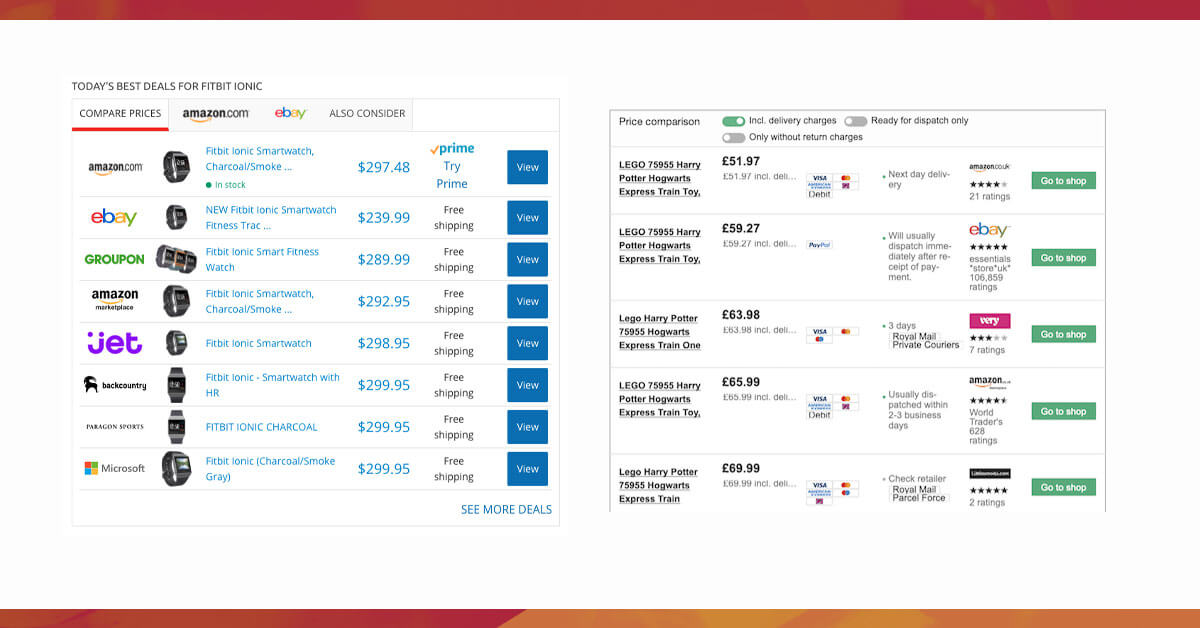**Detailed Caption:**

This image is a comparison snapshot of today's best deals for the Fitbit Ionic, presented in two distinct segments. The left section features a highlighted "COMPARE PRICES" header in red, indicating the selected view. This section lists Fitbit Ionic deals from various retailers including Amazon.com, eBay, Groupon, Amazon, Jet, a company starting with 'B' (likely Back something), an indistinguishable company due to small text, and Microsoft. It displays details such as the availability, pricing, shipping options (Prime, Try Prime, or Free Shipping), and includes a "View" link in a darker blue color along with a "See More Deals" option.

On the right, the section is primarily focused on price comparison and includes filters with toggled options for "Included Delivery Charges" (green, toggled on), "Ready for Dispatch Only" (toggled off), and "Only Without Return Charges" (toggled off). The price comparison listed under this segment includes vendors such as Amazon, eBay, Very, another instance of Amazon, and an unidentified company encased in a black rectangle. It displays prices in GBP, unlike the USD prices on the left. An example product name shown here is "Lego 75955 Harry Potter Hogwarts Express Train Toy". Green "Go to Shop" buttons line the far right of this section.